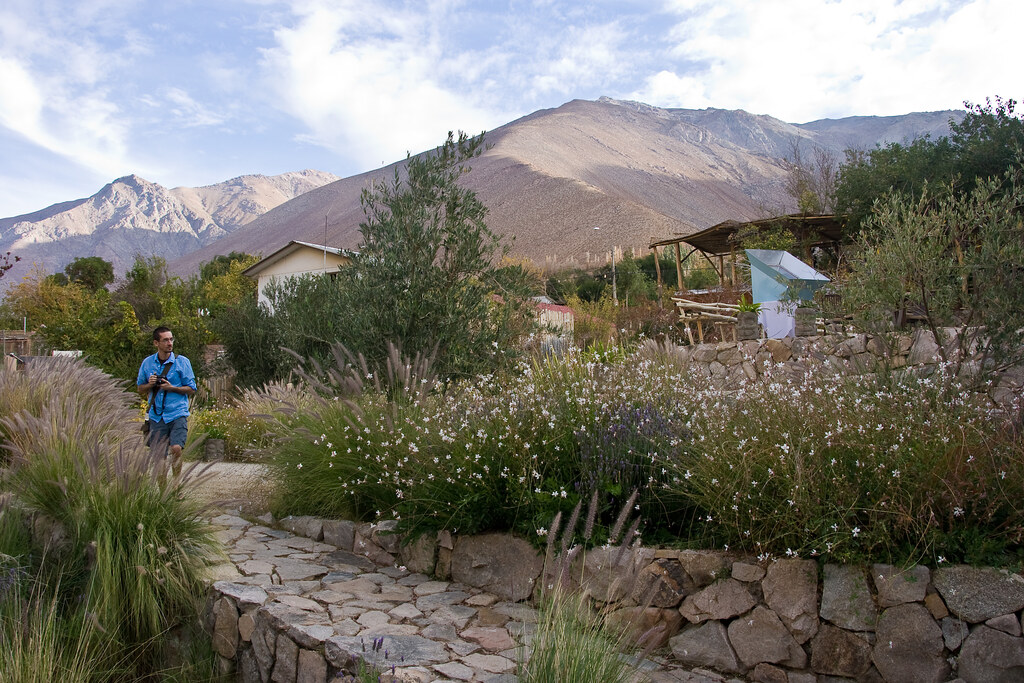The photograph captures a striking outdoor scene featuring barren, rocky mountains in the background. The mountains are primarily brown and dirt-covered, although the furthest peak appears to have a dusting of snow. In the foreground, a stone cobblestone path leads towards a white house partially obscured by a tree or bush. The path is flanked by overgrown grassy plants and white flowers, creating a vibrant contrast to the arid landscape. Along this path, a man with short brown hair, glasses, and a black camera strap across his chest is seen walking. He is dressed in a bright blue short-sleeved shirt and blue shorts. The scene also includes a wooden structure near the house, adding to the rustic charm of this secluded trail.